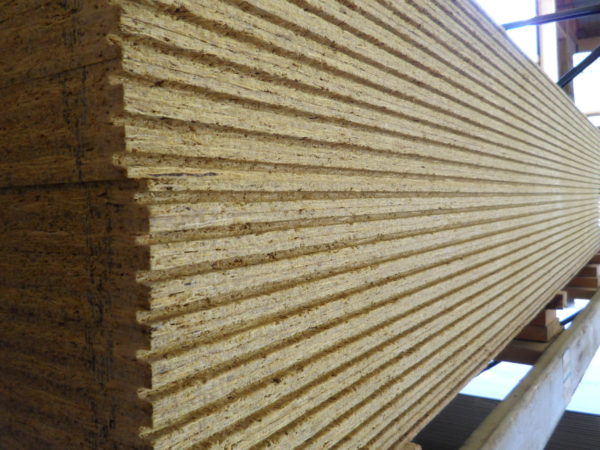This image depicts a close-up and side profile view of a stack of wood planks, likely OSB (Oriented Strand Board) sheets, arranged on a wooden pallet within a lumberyard setting. The wood appears light tannish-brown and features a mottled grain, typical of particle boards. The planks are stacked approximately 20 layers high, with vertical grooves visible, and are supported by 2x4s underneath. The left side of the wood stack is shrouded in shadow, while sunlight filters through the background, suggesting the setting is partially covered yet exposed to a sunny day. The environment gives hints of a warehouse-like structure, with a mix of wood and possible metal components at one end, and overall, the focus remains on the intricate textures and colors of the wood against a simple backdrop.